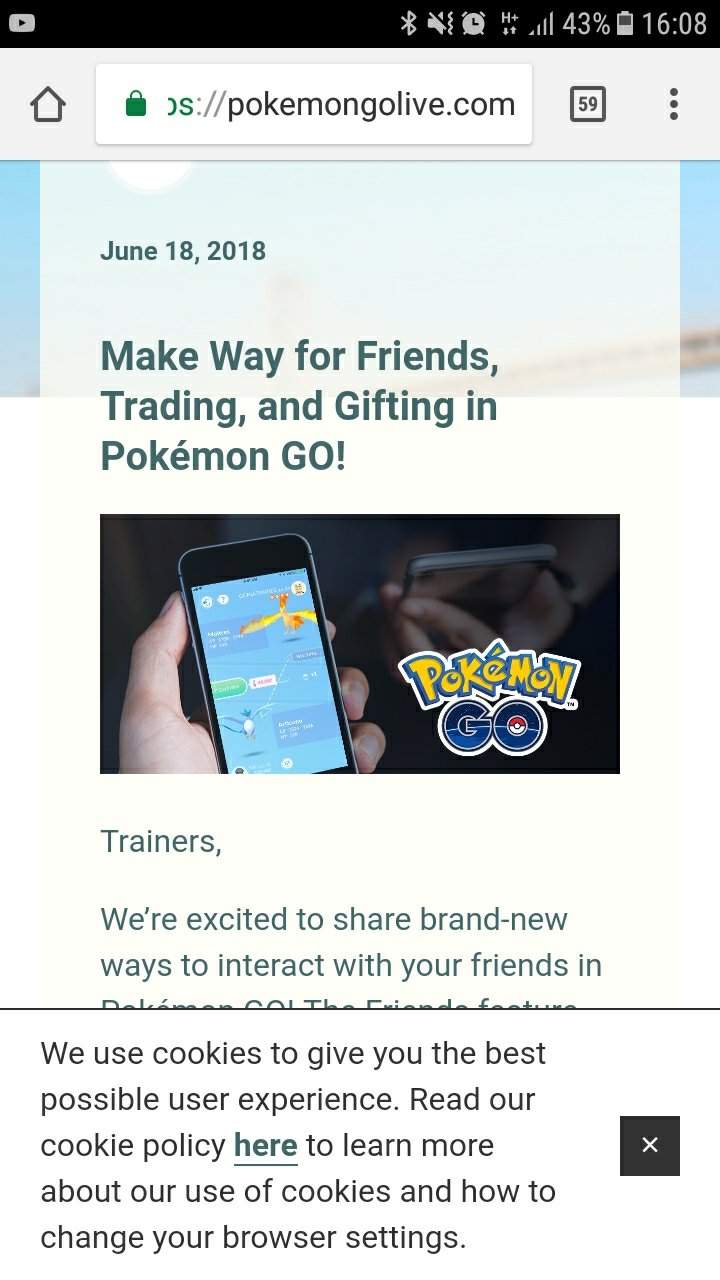In this image, captured as a screenshot from a smartphone, several distinct details are visible. At the top right, the current time is displayed as 16:08. Next to the time, a battery icon indicates a 43% charge, and to its left, the full bars of the phone signal strength are shown. Additionally, there are icons for an alarm clock, a sound icon that is crossed out (suggesting the phone is on silent), and a Bluetooth symbol. On the top left corner, a YouTube icon is seen.

In the main content area of the screenshot, the URL bar reads "PokemonGoLive.com," with a square to the right showing the number 59, indicating the number of open tabs in the browser. The central portion of the screen prominently features the text "Make way for friends, trading and gifting in Pokémon Go," alongside an image of a person holding a phone displaying the Pokémon Go app. Below this image, there's a message that begins with "Trainers, we're excited to share brand new ways to interact with your friends in Pokémon Go."

At the bottom of the image, a pop-up notification reads: "We use cookies to give you the best possible user experience. Read our cookie policy here to learn more about our use of cookies and how to change your browser settings." This thorough description encapsulates the various elements present in the screenshot.